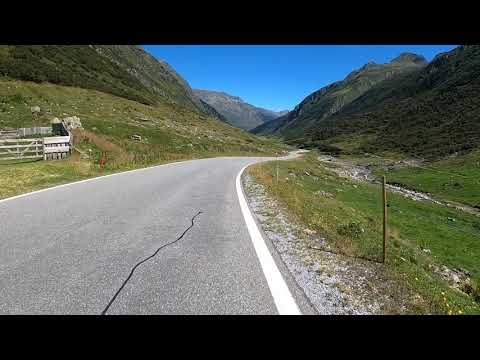The photograph captures a single-lane, light gray asphalt country road meandering through a verdant mountainous landscape. The road, bordered by white lines at its edges, begins in the bottom left corner of the frame and extends upward, vanishing into a gap between the lush, tree-covered mountains. A noticeable crack runs down the center of the well-maintained road. On either side, short, well-kept grass flanks the road, and in the immediate foreground on the left stands an old wooden fence, suggesting an aged horse pen or enclosure without a roof. The scene is bathed in sun with a clear, cloudless blue sky visible between the mountains, emphasizing the rural, tranquil setting. No cars or people are present, adding to the serene, remote atmosphere of this picturesque mountain road.